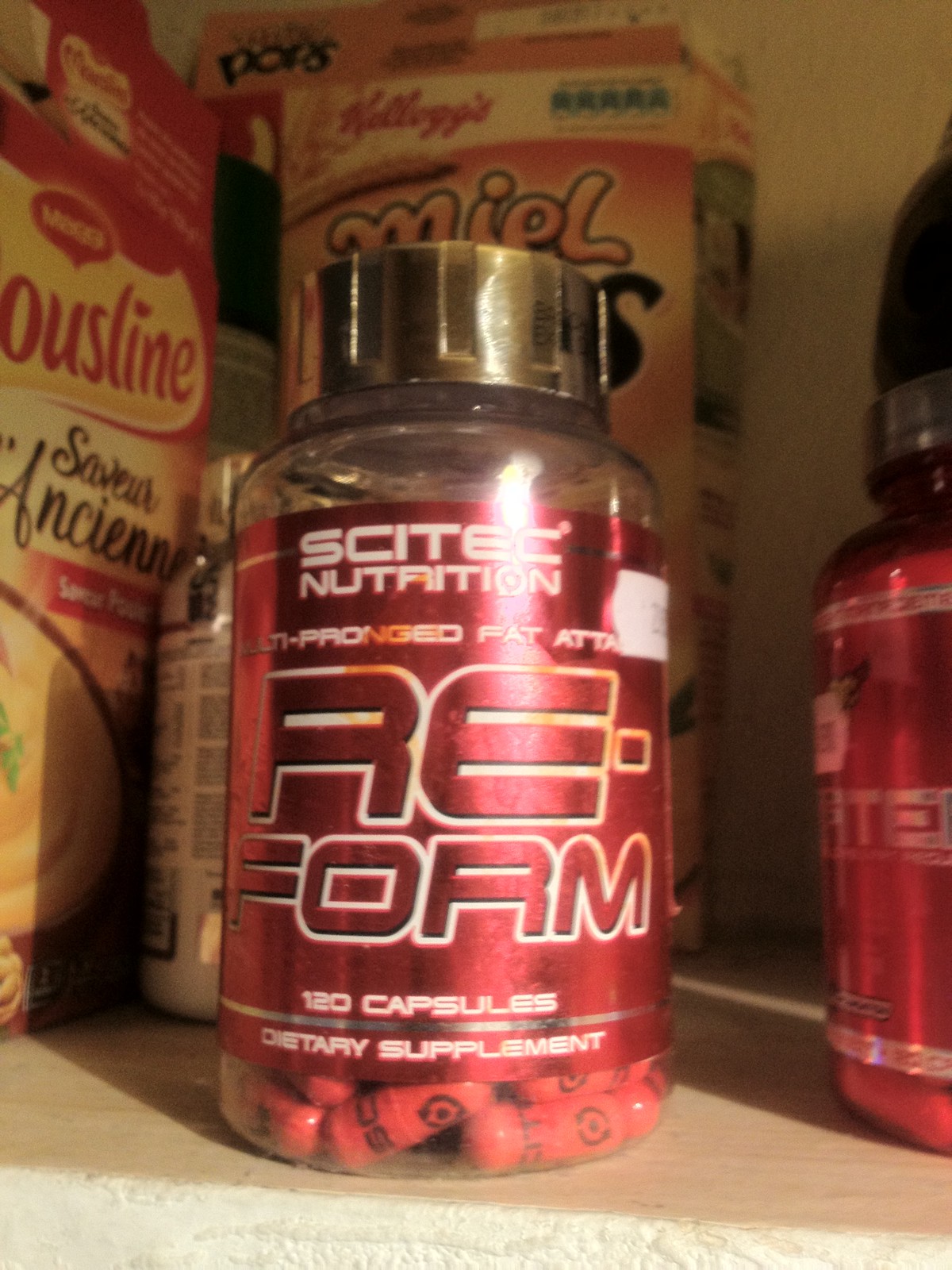In this indoor photo, a wooden shelf holds two plastic bottles of dietary supplements prominently in the foreground. Each bottle by Cytec Nutrition is labeled "Reform" and contains 120 red capsules with black writing, denoted as a "Multi-Pronged Fat Attack" supplement. The bottles feature a red and silver label, and each bottle is capped with a silver-colored top. In the background, there are two cardboard boxes; the one on the left features writing in a foreign language, while the two at the back are Kellogg's Pop cereal boxes. The shelf, reminiscent of a cupboard or pantry setting, underscores the casual storage of these items.